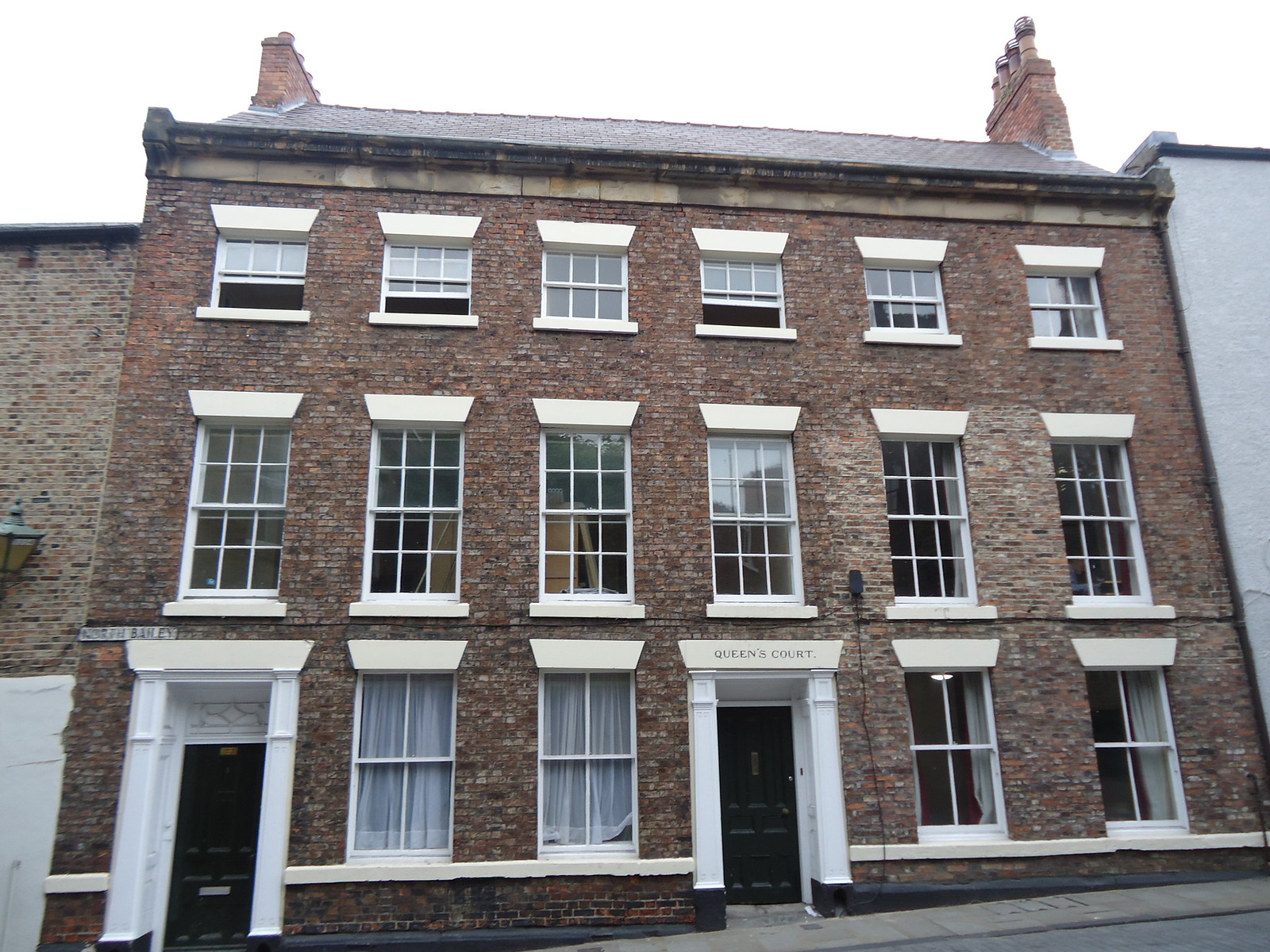This photograph captures an elegant and historical building named Queen's Court, situated in Durham, England. The three-story structure, built from light red brick, exudes a distinct character reminiscent of early 20th or late 19th-century architecture. The building's symmetrical façade features several double-hung windows, each encased in white and adorned with cream-colored decorative ledges above. The ground-floor windows are larger, creating a balanced and inviting appearance.

Queen's Court has two prominent black doors; the central entrance is especially notable with its sign above it declaring the building's name. This doorway is flanked by white pillars, adding an air of grandeur. Another black door is positioned to the left of the central one, enhancing the building's symmetrical design.

The roofline is punctuated by chimneys on both the right and left sides, contributing to the classic architectural style. The gutters along the roof appear aged, matching the vintage aesthetic of the structure. The streets and sidewalks in front of Queen's Court are possibly made of brick, reinforcing the historical ambiance of the locale. Although adjacent buildings are not visible in the photograph, the description indicates they are closely packed, with one being white and the other made of brick. This detailed context further situates Queen's Court within a historic and densely built environment.